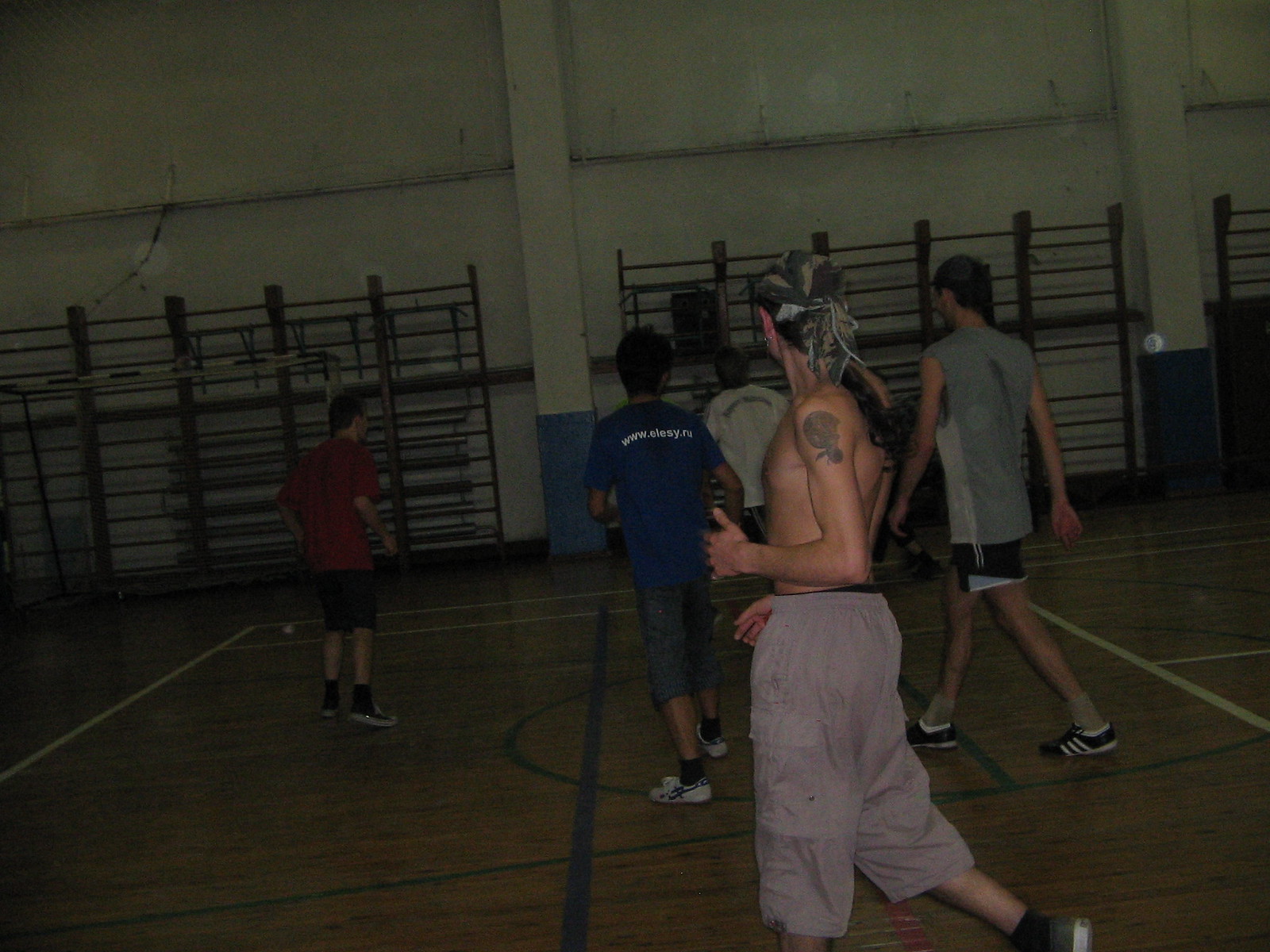The photograph depicts a dimly lit indoor gymnasium, featuring a wooden basketball court marked with blue and white lines. The gym's white walls are accented with brown wooden racks and folded grandstands against one side. Prominently, a shirtless young man with long, purple shorts nearly reaching mid-calf stands closest to the camera. He has a distinctive rose tattoo on his left shoulder and intricately braided hair with highlights, slightly turning his head. Ahead of him, five other young men with their backs to the camera walk towards the back wall, each donned in varying colored shirts and shorts. The faint lighting and the collective movement towards the wall add a dynamic, almost contemplative atmosphere to the scene.